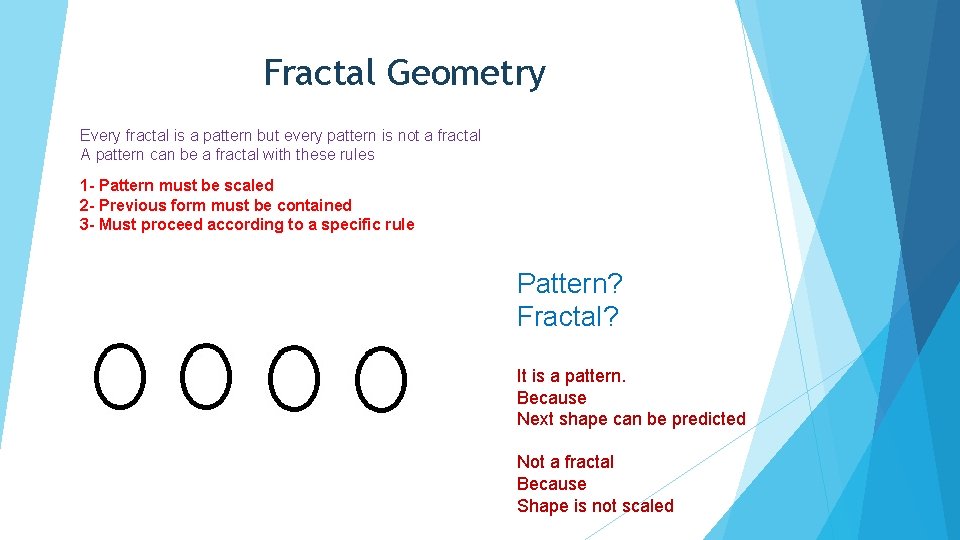This image, possibly a page from a math book or a mathematical advertisement card, is titled "Fractal Geometry" in dark blue text at the top center. Below this title, purple text states, "Every fractal is a pattern but every pattern is not a fractal." It further explains, "A pattern can be a fractal with these rules," followed by three rules in bold red text: "1. Pattern must be scaled," "2. Previous form must be contained," and "3. Must proceed according to a specific rule."

Beneath these rules are four egg-shaped designs with white fills and black outlines. To their right, in blue text, are the words "Pattern?" and "Fractal?" Underneath this, a bold red text explains, "It is a pattern because next shape can be predicted" and "Not a fractal because shape is not scaled." To the right, a geometric design featuring various shades of blue transitioning to white suggests examples of fractals. The overall layout uses a white background and integrates red, black, and blue elements to highlight different aspects of fractal geometry and pattern differentiation.